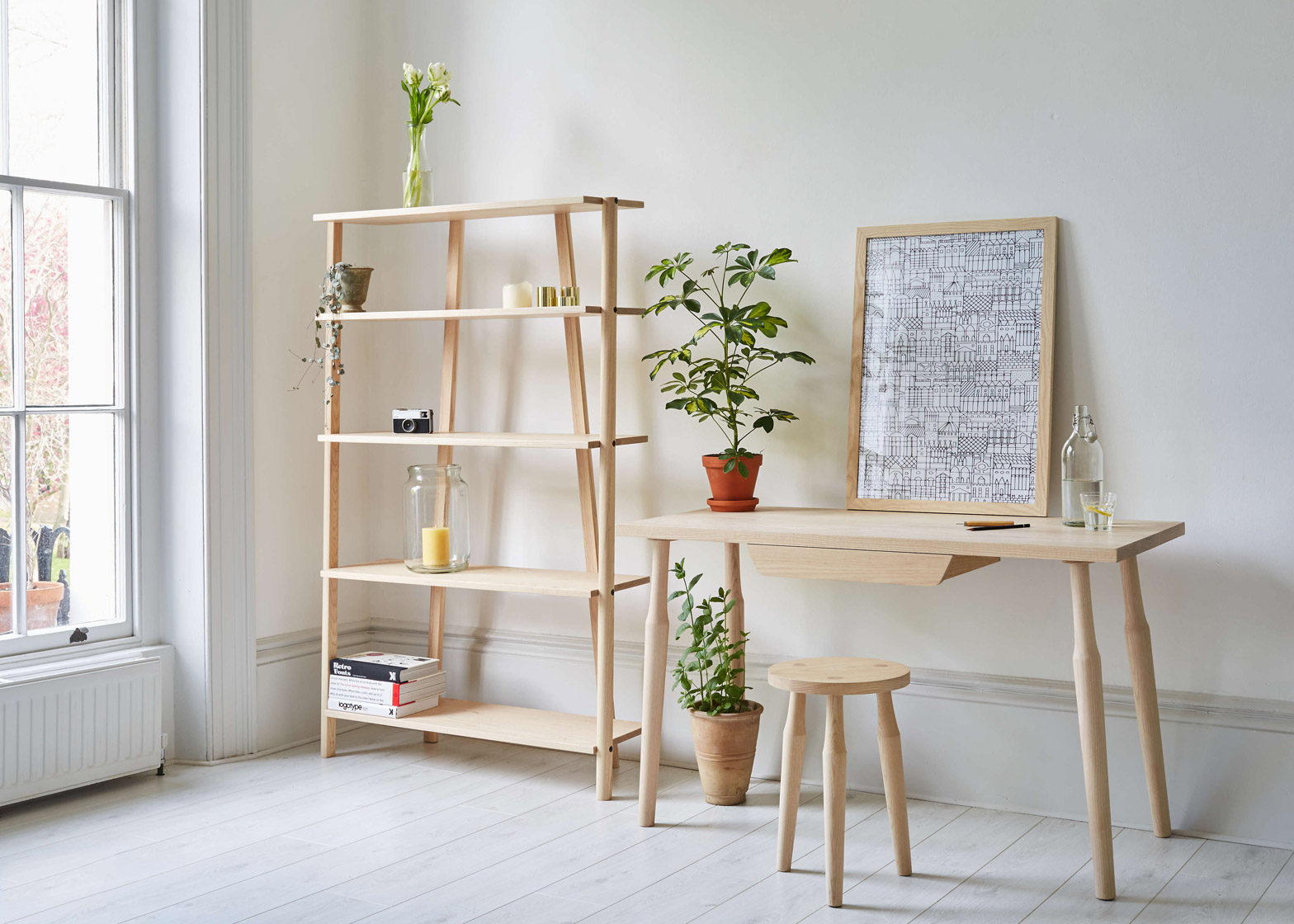The image depicts a minimalist home studio room bathed in white, featuring light-colored wood furnishings. Dominating the left side is a large window without curtains, under which sits a white radiator. Adjacent to this is a wooden shelf unit with five tiers: the bottom shelf holds a collection of books, the next shelf up houses a large glass container with a candle inside, above that is an old camera, followed by a small bowl with a trailing plant, and the top shelf secures a vase with flowers.

To the right of the shelf stands a simple light brown wooden desk paired with a matching barstool. The desk has a central drawer and displays a few items: a bottle filled with water, a glass, a pencil, and a pen. At the desk's left edge sits a potted water plant, and another potted plant rests on the floor beneath it. Above the desk, pinned on the wall, is a poster featuring a complex black-line diagram on a white background. The entire room exudes a clean, minimalist aesthetic with its plain white walls and floor.